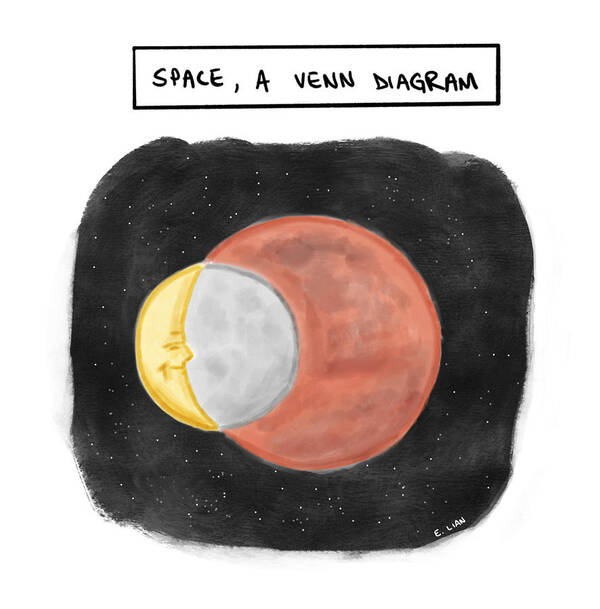The painting features a black nighttime sky, loosely defined by a horizontal rectangle, sprinkled with white speckles resembling stars. At the center of this black background is a dull, pinkish-red sphere outlined in a darker reddish hue, representing a planet. To the left of the planet, a distinctive crescent moon with a smiling face, eyes closed and eyebrows visible, overlays the red sphere. The crescent is golden, while the rest of the moon is light gray, outlined in dark gray. Above this celestial scene, in a white horizontal rectangle bordered by a black line, is handwritten text in all caps: "SPACE, A VENN DIAGRAM." The artwork's style suggests a blend of watercolor and acrylic paints, contributing to its muted tone. In the bottom right corner of the black sky area, the signature "E. LIAN" is marked, accompanied by stars around it. The illustration combines artistic representations of the moon, the planet, and the concept of space, though the precise relation to a Venn diagram remains abstract.